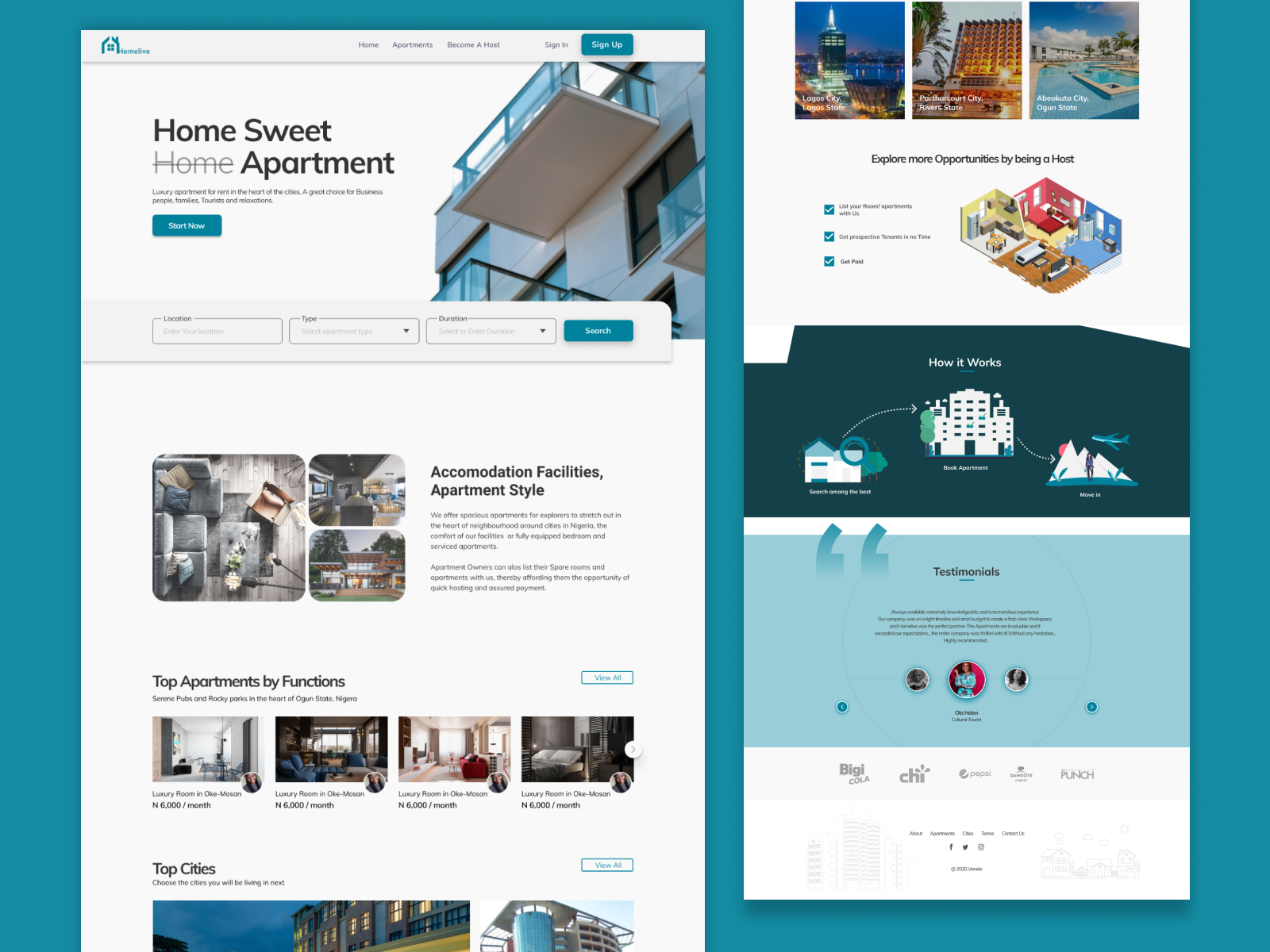The image showcases a welcoming home rental platform offering various property listings including home suites, apartments, and luxury apartments for rent in prime city locations. The website features easy navigation with options to become a host, sign in, or sign up. It caters to business professionals, families, and tourists seeking comfort and relaxation. Detailed prompts encourage users to explore hosting opportunities, list their properties, attract potential tenants quickly, and earn rental income seamlessly.